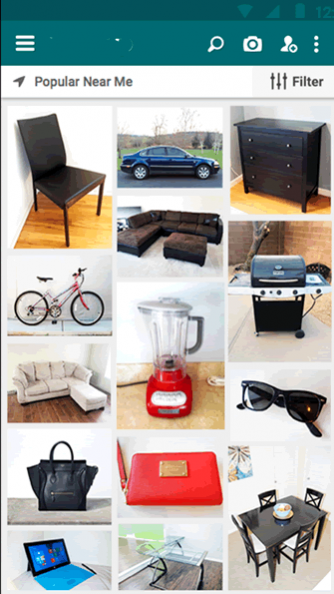The image appears to be a screenshot of a mobile app interface, captured on someone's phone. The top section of the app is dark teal in color, featuring several white icons. On the far left, there are three horizontal lines, commonly representing a menu. Next to it is a white magnifying glass icon for search functionality, followed by a white camera icon. Adjacent to the camera icon is a white outline of a person with a plus symbol, suggesting the option to add or follow users. There are also three small white circles aligned horizontally.

Below this dark teal section, the background transitions to an off-white color, prominently displaying the title "Popular Near Me" in gray text. Immediately below the title, there's an option labeled "Filter".

The main content area contains a grid of images organized into three columns, showcasing various items. From top to bottom, the first column includes:
1. A black chair.
2. A bike that appears to be silver and pink.
3. A white sectional sofa.
4. A black pocketbook.
5. A black tablet.
6. A black car.

The second column features:
1. A brown sectional sofa.
2. A red blender.
3. A red bracelet with gold accents.
4. A clear glass table with a wooden surface.
5. A brownish-black wooden dresser with three rows of shelves.
6. A black and silver metal grill.

The third column displays:
1. A pair of black glasses on a white surface.
2. A dark brown or black rectangular dining room table situated on a beige carpet.

Each item is presented as an image in a neat and elongated rectangular format, making the interface visually organized and user-friendly.